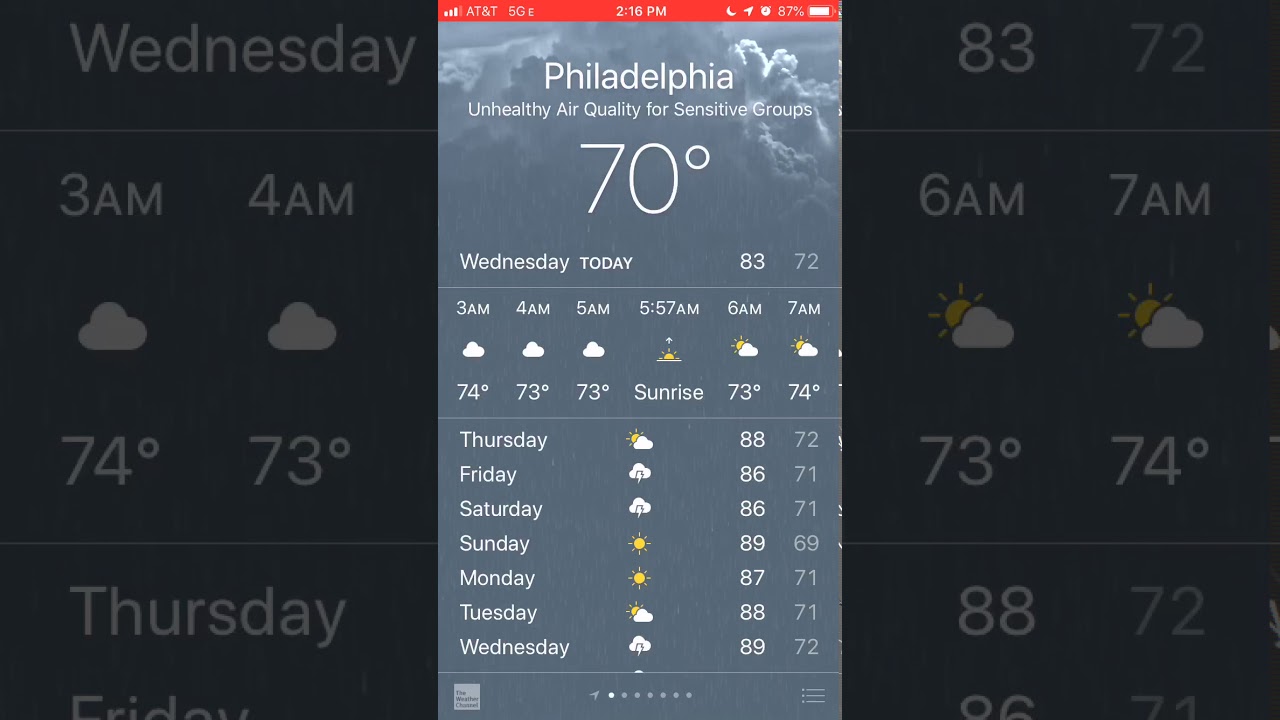This screenshot captures a moment from a phone screen recording, indicated by the red bar at the top of the screen. The device is connected to AT&T's 5G network, showing three out of four bars for signal strength. It is 2:16 p.m., and the phone is in "Do Not Disturb" mode, as noted by the crescent moon icon. The presence of the location symbol suggests a location-tracking service is active, and an alarm is set, evidenced by the alarm clock icon. The battery level of the phone is at 80%.

The phone's screen displays the weather app focused on Philadelphia. The current temperature is 70°F with a warning about "Unhealthy Air Quality for Sensitive Groups." The forecast also details the day's high of 83°F and a low of 72°F. Specific hourly predictions include:

- 3 a.m.: 74°F
- 4 a.m.: 73°F
- 5 a.m.: 73°F (sunrise at 5:57 a.m.)
- 6 a.m.: 73°F
- 7 a.m.: 74°F

The app further displays the extended forecast for the upcoming days:
- **Thursday**: Partly cloudy, high of 88°F, low of 72°F.
- **Friday**: Thunderstorms and rain, high of 86°F, low of 71°F.
- **Saturday**: Thunderstorms and rain, high of 86°F, low of 71°F.
- **Sunday**: Sunny, high of 89°F, low of 69°F.
- **Monday**: Sunny, high of 87°F, low of 71°F.
- **Tuesday**: Partly cloudy, high of 88°F, low of 71°F.
- **Wednesday**: Thunderstorms and rain, high of 89°F, low of 72°F.

At the bottom of the screen, there are seven navigation options available, allowing the user to switch between saved locations for different weather forecasts.